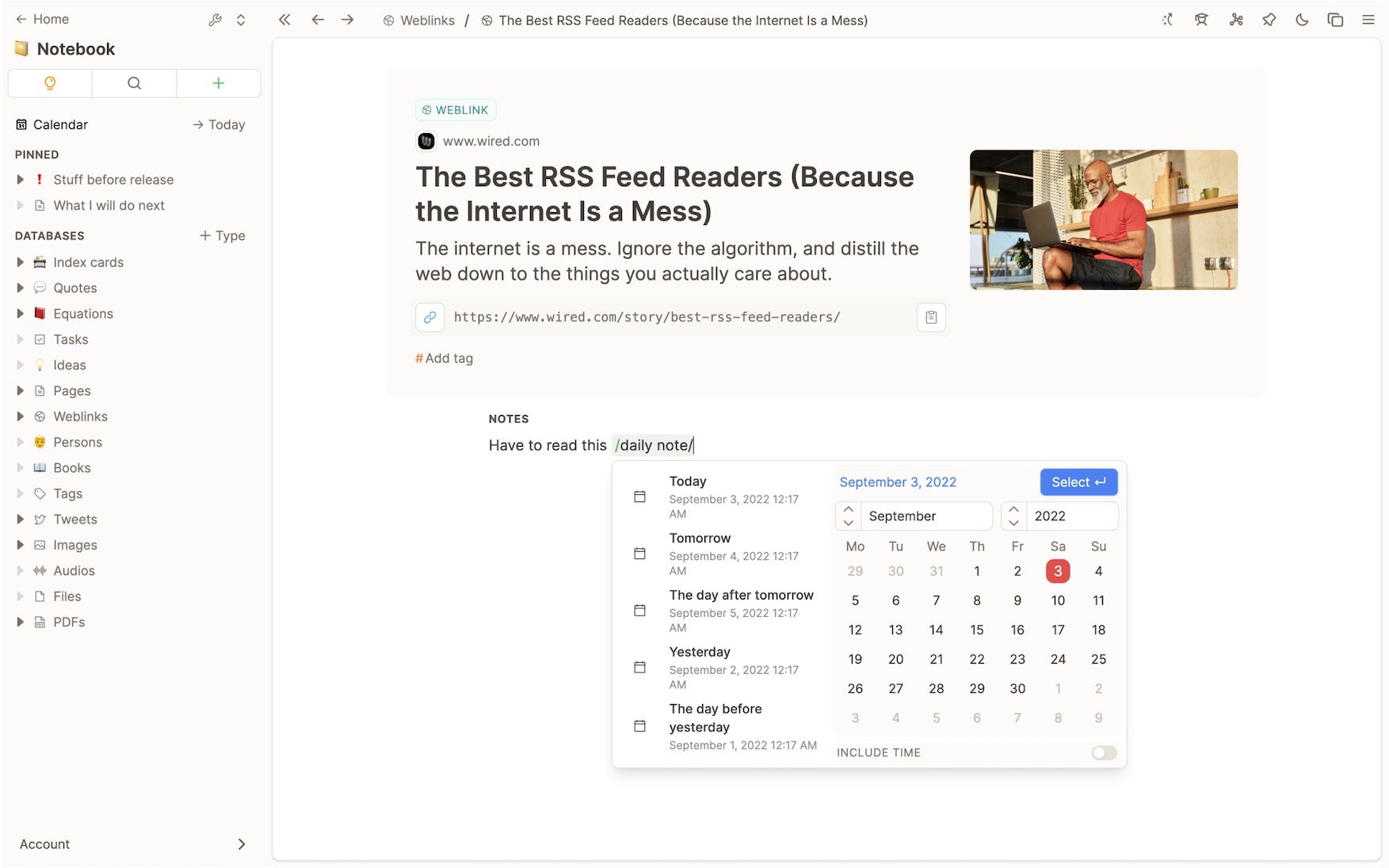The image depicts a digital Notion notebook interface. At the top, there's a navigation menu listing sections such as "Home," "The Notebook," "Calendar," "Today," "Pinned," and "Stuff for Release." Another section titled "What I Will Do Next" follows. Below this, a variety of database links are listed, including "Index Cards," "Quotes," "Equations," "Tasks," "Ideas," "Pages," "Web Links," "Persons," "Books," "Text," "Tweets," "Images," "Audios," "Files," and "PDFs."

At the very top, navigation arrows (left and right) are visible, alongside symbols for a web link and a slash. The main content area displays two web links: "The Best RSS Feed Readers (Because the Internet is a Mess)" twice, emphasizing the theme that the internet is cluttered and advocating for a curated feed experience. The content urges users to "Ignore the algorithm and distill the web down to things you actually care about."

There is also a note attributed to "Wired," followed by various snippets and dated notes, such as "How to Read This," "Daily Note," "Today," "Tomorrow," with specific dates for clarity. The current day is marked as "Today is September 3rd, 2022," and subsequent days follow in order.

Moreover, a calendar shows September 2022, with September 3rd highlighted both in blue and red, marking it as the selected date.

This saved page seems to be a detailed overview and endorsement for using RSS readers for a more streamlined internet experience.